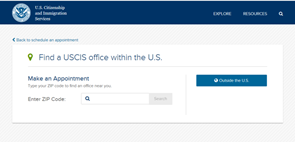The website graphic features a dark blue banner at the top, prominently displaying a round emblem on the left. The emblem contains blurred text in white that reads "U.S. Citizenship and Immigration Services". To the right, the banner has the words "Explore" and "Resources", accompanied by a white magnifying glass icon.

Beneath the banner, the header transitions into a gray background that includes a right-facing arrow icon with the text "Back to Schedule an Appointment". Below this, there is a prominent white square.

At the top of the white square, a green heading announces "Find a USCIS Office within the U.S.", with "USCIS" fully capitalized. A thin line separates this heading from the subsequent text below.

Further down, the text "Make an Appointment" appears in dark blue, with both the "M" and "A" capitalized. Directly underneath, instructions in black state, "Type your ZIP Code to find an office near you."

Below these instructions is a labeled input field that reads "Enter your ZIP Code", with "ZIP" and "Code" both capitalized. This field is followed by a "Search" button featuring a magnifying glass icon.

Adjacent to this, a blue, clickable button labeled "Outside the U.S." provides an option for users seeking international locations.